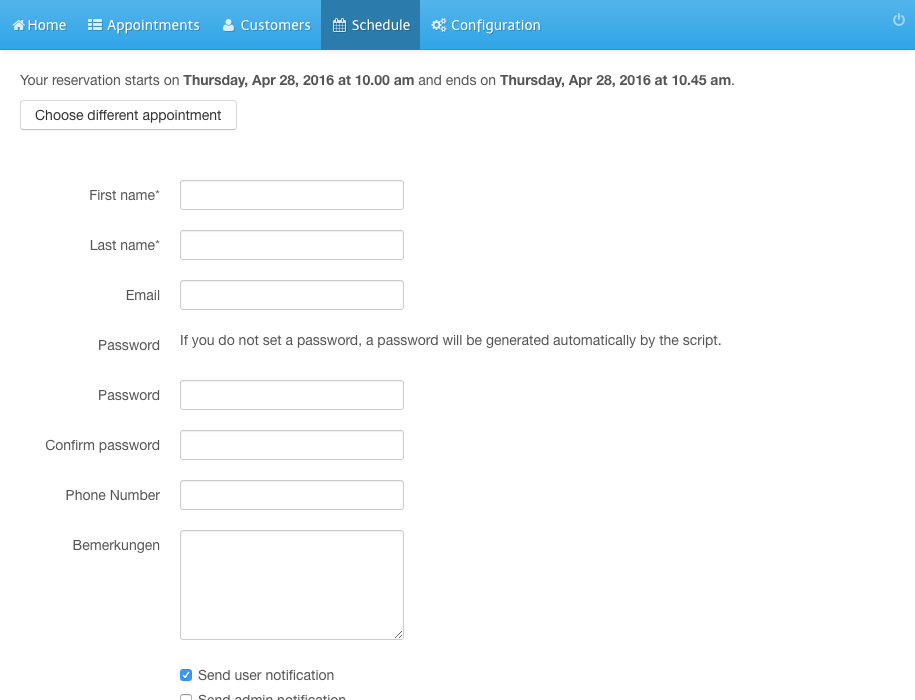The image is a detailed screenshot of a website's schedule form. At the top of the screenshot is a blue navigation bar featuring a variety of clickable tab options. Starting from the left, there is a "Home" button accompanied by a small house icon. Moving rightward, the options include "Appointments" marked with dashes and dots, "Customers" symbolized by a person icon, "Schedule" represented with a calendar icon, and "Configuration" indicated by three gear symbols. Positioned in the upper right-hand corner of the bar is a Power button.

Below this navigation bar, text states that a reservation starts on Thursday, April 28, 2016, at 10 AM and ends on the same day at 10:45 AM. Below this information, there is a clickable button labeled "Choose Different Appointment."

Beneath this button is a form designed to collect various pieces of information from the user. The form consists of the following input fields:
- First Name: A text box is provided.
- Last Name: A text box is provided.
- Email: A text box is provided.
- Password: It includes a notice that if no password is set, one will be generated automatically by the script.
- Confirm Password: A text box is provided for confirmation.
- Phone Number: A text box is provided.
- A German word, "Bemerkunden," followed by a very large text box which likely stands for additional comments or remarks.

At the bottom of the form, there are options for notifications. Users can check "Send User Notification" (currently checked) and "Send Admin Notification," although the latter is partially cut off in the screenshot.